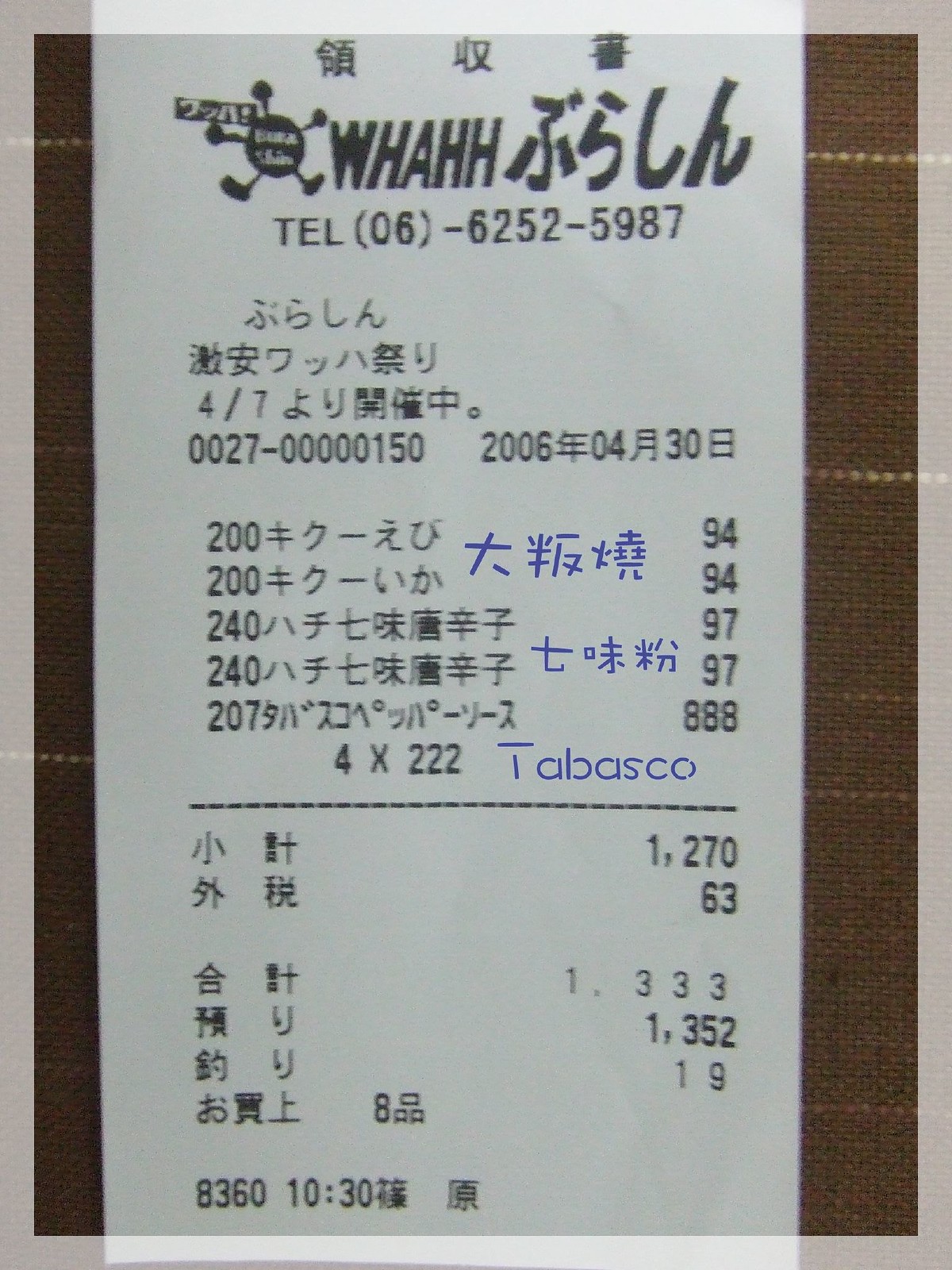A detailed caption for the image could be:

"A crumpled receipt from the restaurant Wa-Ha-Ha, resting on a brown fabric background. The receipt features a mix of printed and handwritten elements. There are Asiatic characters, likely indicating it is from a non-American establishment, along with a non-American telephone number. The date is not legible. In black ink, it lists five purchases with the total amount being 1,352. There are also blue handwritten characters on the receipt and the word 'Tabasco' is visibly written. A mysterious symbol appears to the left of the text. The transaction occurred at 10:30, though it's unclear whether it was in the morning or afternoon."